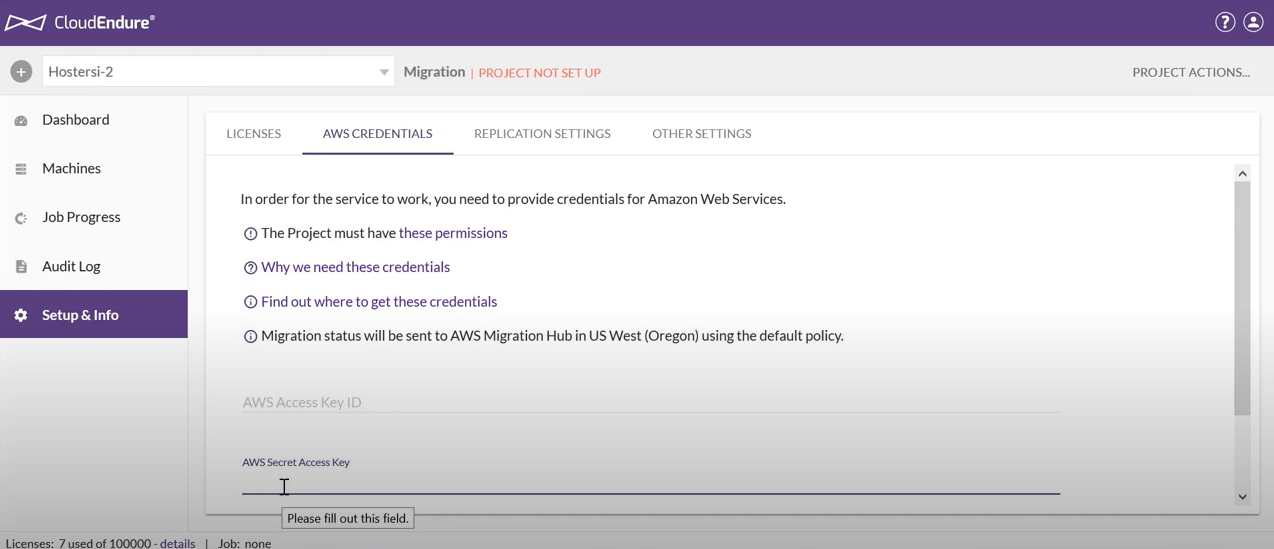This screenshot captures a cropped image of a webpage with a predominantly light purple background. The top banner, dark purple in color, prominently displays the "CloudEndure" text and logo on the left in white. To the right of the banner, there are icons for help (a question mark) and user account settings (an account icon).

Below the top banner, the body of the webpage also features a light purple background. In the upper left corner, there is a dropdown box with a plus sign to its left. To the right of the dropdown box, "Migration" is displayed, followed by "Project Not Setup" in red letters, indicating an incomplete setup status.

A left-hand panel beneath this header contains navigation options, such as Dashboard, Machines, Job Progress, Audit Log, and Setup and Info. The option "Setup and Info" is highlighted in dark purple, signifying it is currently selected. 

To the right of this panel, the "Setup and Info" section is expanded, displaying several top categories including Licenses, AWS Credentials, Application Settings, and Other Settings. The "AWS Credentials" category is selected, revealing further details below. 

The detailed text reads: "In order for the service to work, you need to provide credentials for Amazon Web Services." To facilitate this, several help options are presented, with clickable question mark icons next to explanations such as "the project must have these permissions," "why we need these credentials," and "find out where to get these credentials."

Overall, the screenshot provides a detailed view of the CloudEndure setup interface, indicating incomplete project setup and focusing on the AWS Credentials configuration section.